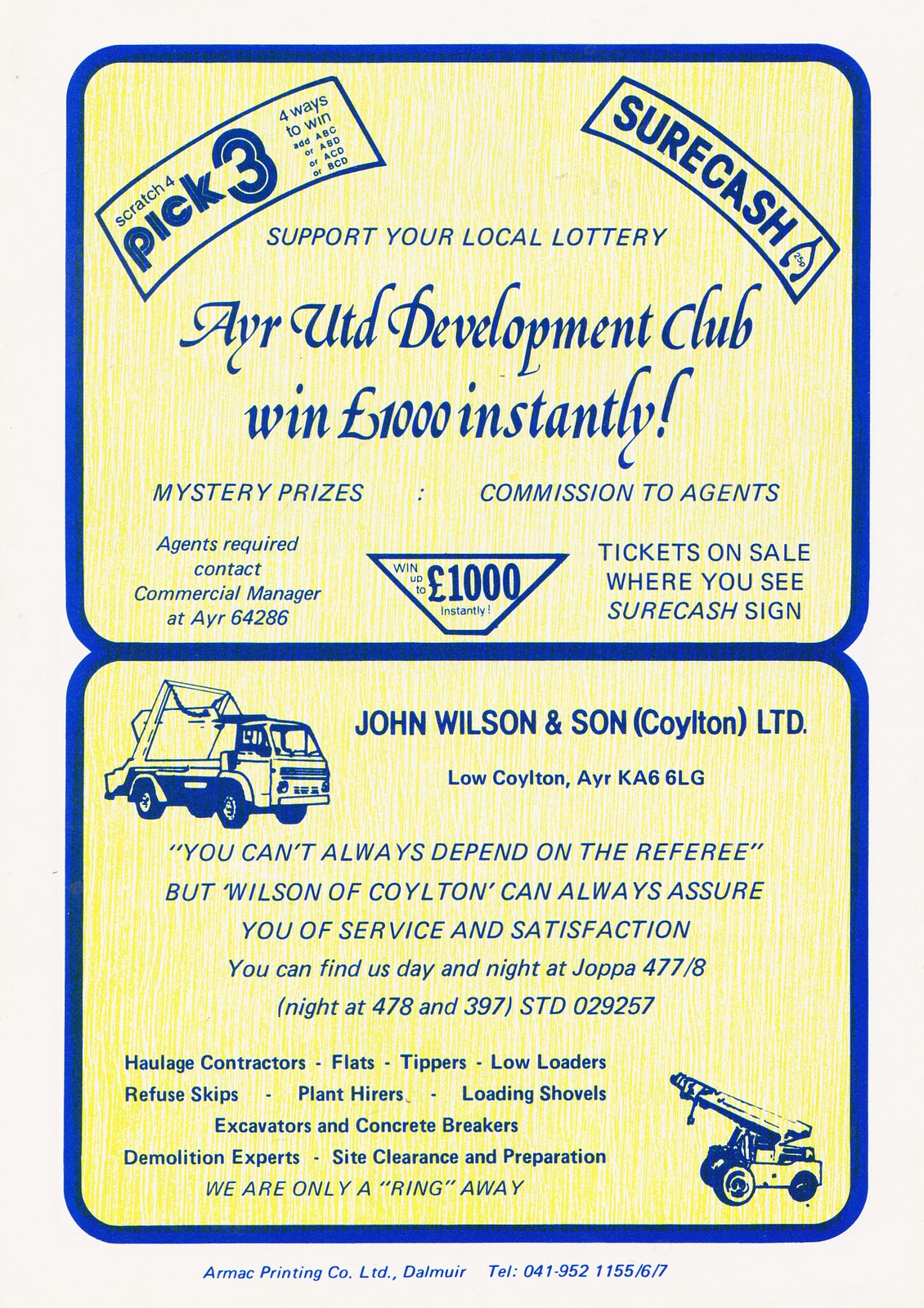The image is a rectangular advertisement divided into two distinct sections, each bordered in a bright royal blue frame against a yellow background, with blue text throughout.

In the top section, the advertisement promotes a local lottery event. It features various boxes and text, including:

- "Scratch for Pick Three, Four Ways to Win" in the top left with a couple of banners.
- "Super Cash" to the right, alongside the text "Support your local lottery AYR UTD Development Club. Win £1000 instantly."
- Additional text reads "Mystery Prizes, Commissioned Agents," and "Agents Required, Contact Commercial Manager at AIR 64286."
- A further detail includes a small rectangle with an upside-down pyramid logo stating "Win up to £1000 Instantly," and a note about tickets being available where the "Super Cash" sign is seen.

The bottom section advertises John Wilson & Son (Coylton) Ltd., a haulage contractor. Key details include:

- The title "John Wilson and Son (Coylton) Limited" with a location at "Loy Coylton, AYR KA66LG."
- A quote: "You can’t always depend on the referee, but Wilson of Coylton can always assure you of service and satisfaction."
- Contact information: "Find us day and night at Joppa 477/8, and night at 478 and 397, STD 02925."
- Services listed: "Haulage Contractors: Flats, Tippers, Low Loaders, Refuse Skips, Plant Hires, Loading Shovels, Excavators, and Concrete Breakers. Demolition Experts, Site Clearance and Preparation. We are only a ring away."
- It also features images, with a dump truck on the left and a crane on the bottom right.

A final detail reads in small blue print: "Our Mac Printing Company Limited. Phone 041-952115/6/7."